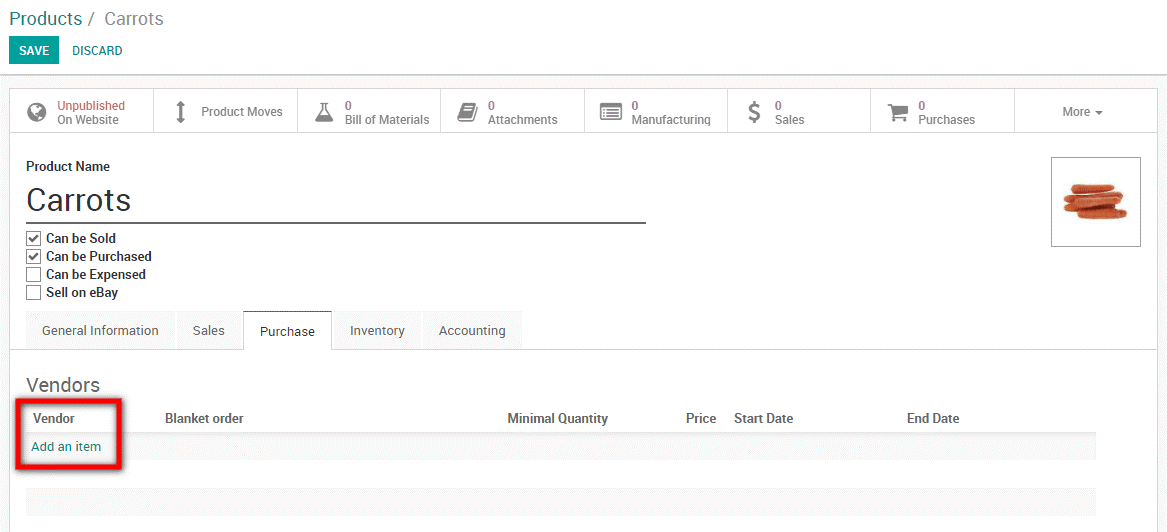The image shows a detailed printout highlighting various aspects of a product listing for carrots. The top section of the printout features a green box with the word "DISCARD" in white print located to the right side, signifying an option to remove the item. Moving from left to right, the page is divided into sections with labels such as "Unpublished on Website," "Product Moves," "Zero Bill of Materials," "Zero Attachments," "Zero Manufacturing," "Zero Sales," and "Zero Purchases," among others.

Below these sections, the product name "Carrots" is prominently displayed. Accompanying this are several options: "Can be Sold," "Can be Purchased," "Can be Expensed," and "Sell on eBay." Check marks are placed in the boxes next to "Can be Sold" and "Can be Purchased," indicating these statuses are active.

Further rows provide tabs labeled "General Information," "Sales," "Purchase," "Inventory," and "Accounting," each potentially leading to more detailed information specific to those categories.

To the right side of the printout, there is an image of five orange carrots neatly placed inside a box. Near the bottom of the page, additional options from left to right are displayed, including "Vendors," "Add Item," "Blanket Order," "Minimum Quantity," "Price," "Start Date," and "End Date."